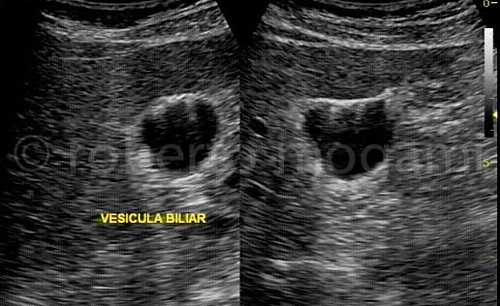The image depicts two side-by-side ultrasound sonograms, commonly performed during pregnancy. Both panels appear almost identical, featuring black and white horizontal lines typical of ultrasound imagery. Prominently, near the center of each panel, there's a notable black area resembling a bear claw. Beneath this black area on the left panel, yellow text spells out "VESICULA BILIAR." Likewise, the right panel features similar black and white wavy lines and an analogous central black area. A watermark reading "Roberto Mon Gummy" in white text is located in the middle of the image. Despite being related to pregnancy ultrasounds, no baby is visible; instead, a sphere-like shape is noticeable in both panels.